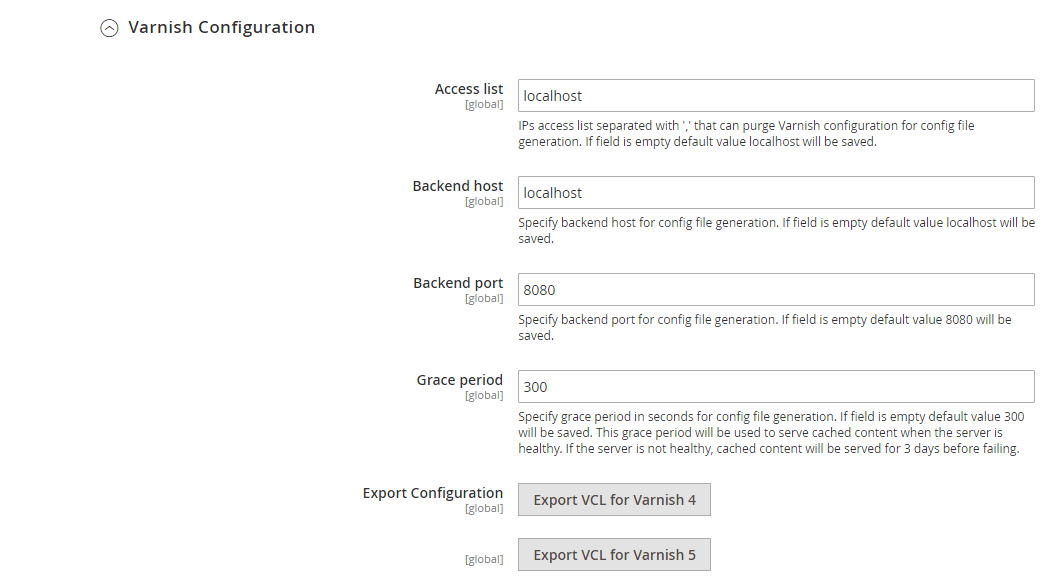The image displays a configuration interface for Varnish with several settings and input fields. In the top left corner, there is a circle with an arrow pointing upwards, labeled "Varnish Configuration." To the immediate right, it is captioned "Access List" with the term "Global" noted underneath in brackets. There is a text box labeled "Local Host," followed by the instruction, "IP Access List Separated."

The interface mentions that users can purge the Varnish Configuration for config file generation if the field is left empty; the default value "Local Host" will be saved. Below this section, it states "Backend Hosts" with "Global" again noted beneath. Here, another text box displays "Local Host," accompanied by instructions to specify backend hosts for configuration file generation. If this field is empty, the default value "Local Host" will be saved.

Further down, there is a section labeled "Backend Port" with "Global" in brackets, and a text box showing the value "8080." Instructions below this text box clarify that users should specify the backend port for config file generation. If the field is empty, the default value "8080" will be saved.

Toward the bottom of the interface, it indicates a "Grace Period" with "Global" in brackets. The corresponding text box displays the number "300," and users are instructed to specify the grace period, in seconds, for config file generation. If this field is left empty, the default value will be used.